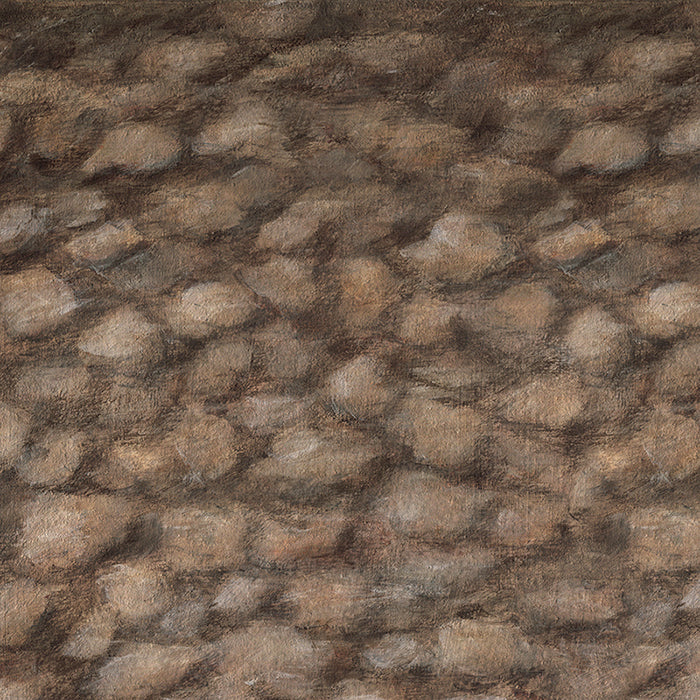The image is a square, highly detailed art piece resembling an oil painting focused on a textured closeup of brown rocks embedded in a riverbed. The composition features a natural color palette dominated by varying shades of brown and tan, with lighter brown lumps and darker lines adding depth and dimension, creating a 3D effect. The rocks appear to be laid flat on a plane, interspersed with brown, mud-like areas, suggesting water running over them and casting intricate highlights and shadows. The top corners of the painting are significantly darker, with the top left being almost blackish, while the bottom left corner is more illuminated, enhancing the impression of dynamic light and movement across the rocky surface.